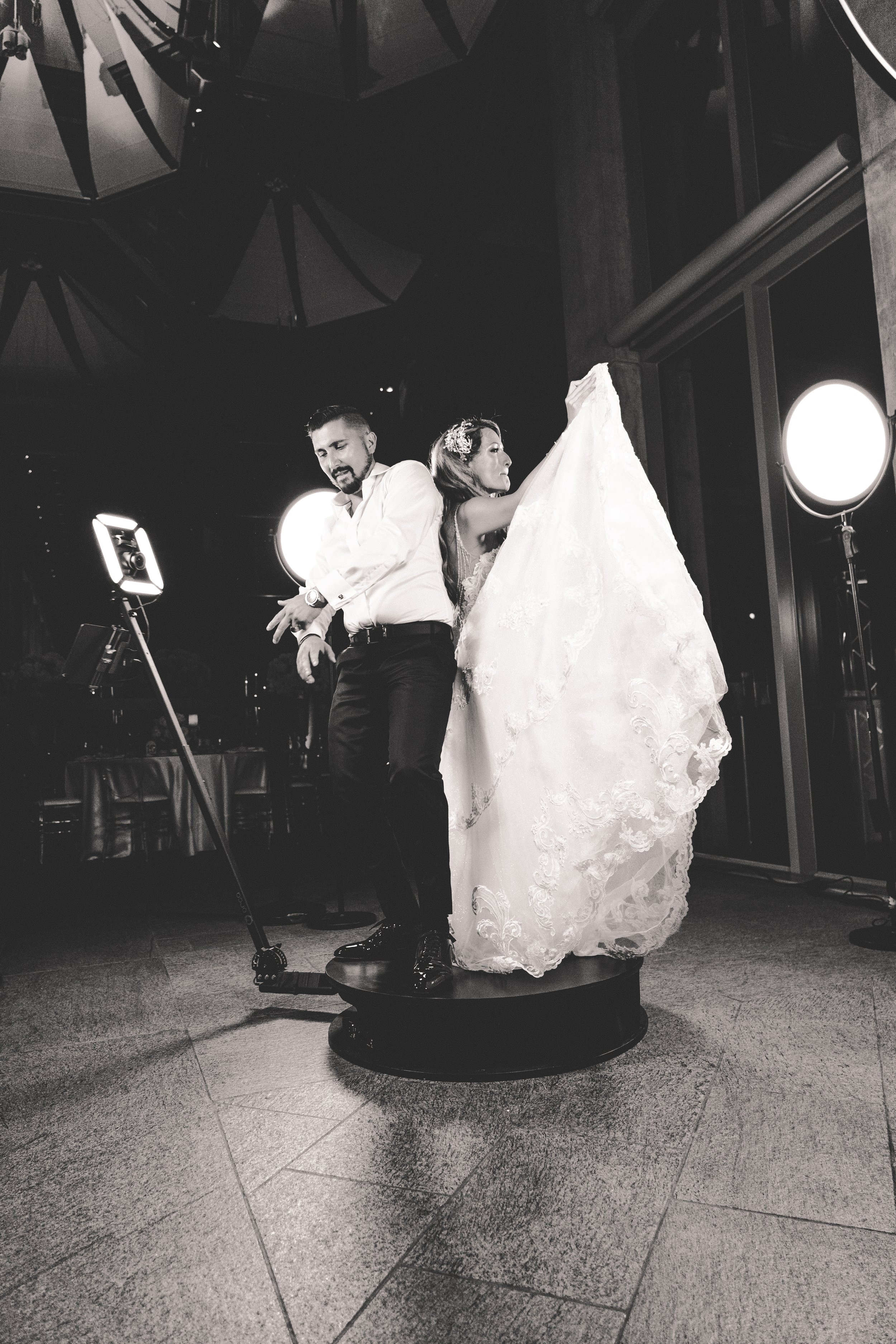In this captivating black and white image, two individuals—presumably newlyweds—celebrate their union. They are standing on a round, rotating platform, engaged in an interactive photo shoot, likely designed to capture their joyous moments from multiple angles. The woman is elegantly dressed in a wedding gown, complete with a fascinator or floral accessory adorning her hair. The man complements her attire with dress slacks and a neatly tucked-in button-up shirt. They are poised away from each other, suggesting the platform's rotation allows them to take turns in front of the camera.

The setting is a meticulously arranged indoor studio with a tiled floor featuring a gray, darker-textured pattern. Illuminating the scene is a square light positioned in front of the couple, while mirror reflections and large windows in the background add depth. Above, numerous lighting umbrellas are suspended from the ceiling, casting a soft, even glow over the scene. The overall atmosphere blends a sense of celebratory intimacy with the sleekness of a professional photo or video shoot.